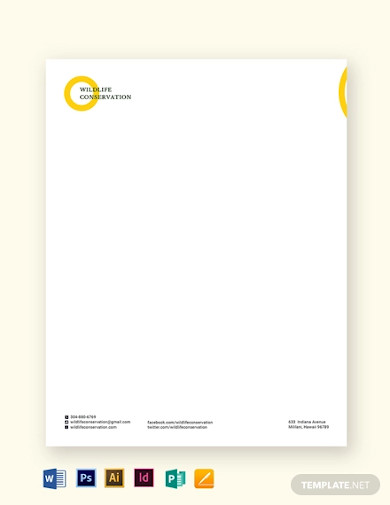The image depicts a blank white rectangle resembling a card or a piece of paper. In the upper left-hand corner, there is a yellow circle with black text next to it that reads "Wildlife Conservation." Adjacent to this, on the top right edge, there is a partial yellow circle that is cut off. At the bottom of the card, centrally aligned and extending slightly to the left and right, there are two to three lines of small black text, which are too minuscule to decipher. Below this text, several icons are visible: a blue square with a white "W" resembling an open book, a black square with "PS" in purple, a brown square with "AI" in yellow, a black square with "ID" in purple, a green icon resembling an open book with a "P," and an orange square with a white pen icon. To the far right of these icons is a gray, rounded rectangle that says "template.net."